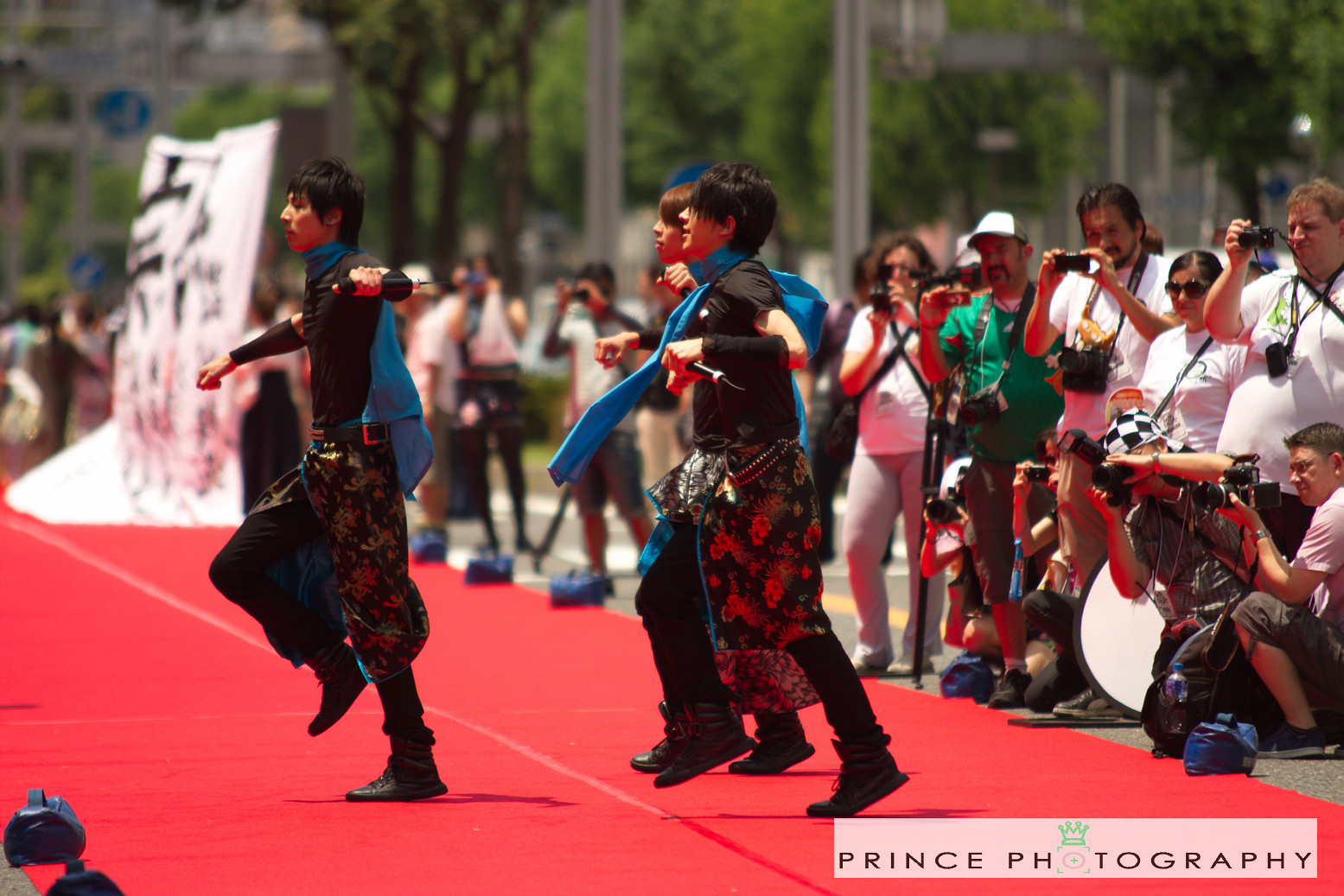This full-color photograph, taken by Prince Photography outdoors on a bright, sunny day, captures a vibrant cultural performance, possibly in the Middle East. In the foreground, three young male dancers, dressed in black t-shirts, red and black pants, black socks, and blue scarves around their necks, execute a traditional dance on a prominent red carpet. Both have their right legs lifted in mid-dance. The red carpet is adorned with several blue spotlights, not in use due to the daylight. Behind the dancers stands a crowd of spectators, many equipped with photo and video cameras, capturing the performance. To the upper left of the image, partially visible, is a large white banner with blurred text, likely describing the festival or ceremony. The backdrop features lush trees and a few poles, enhancing the outdoor setting's charm.